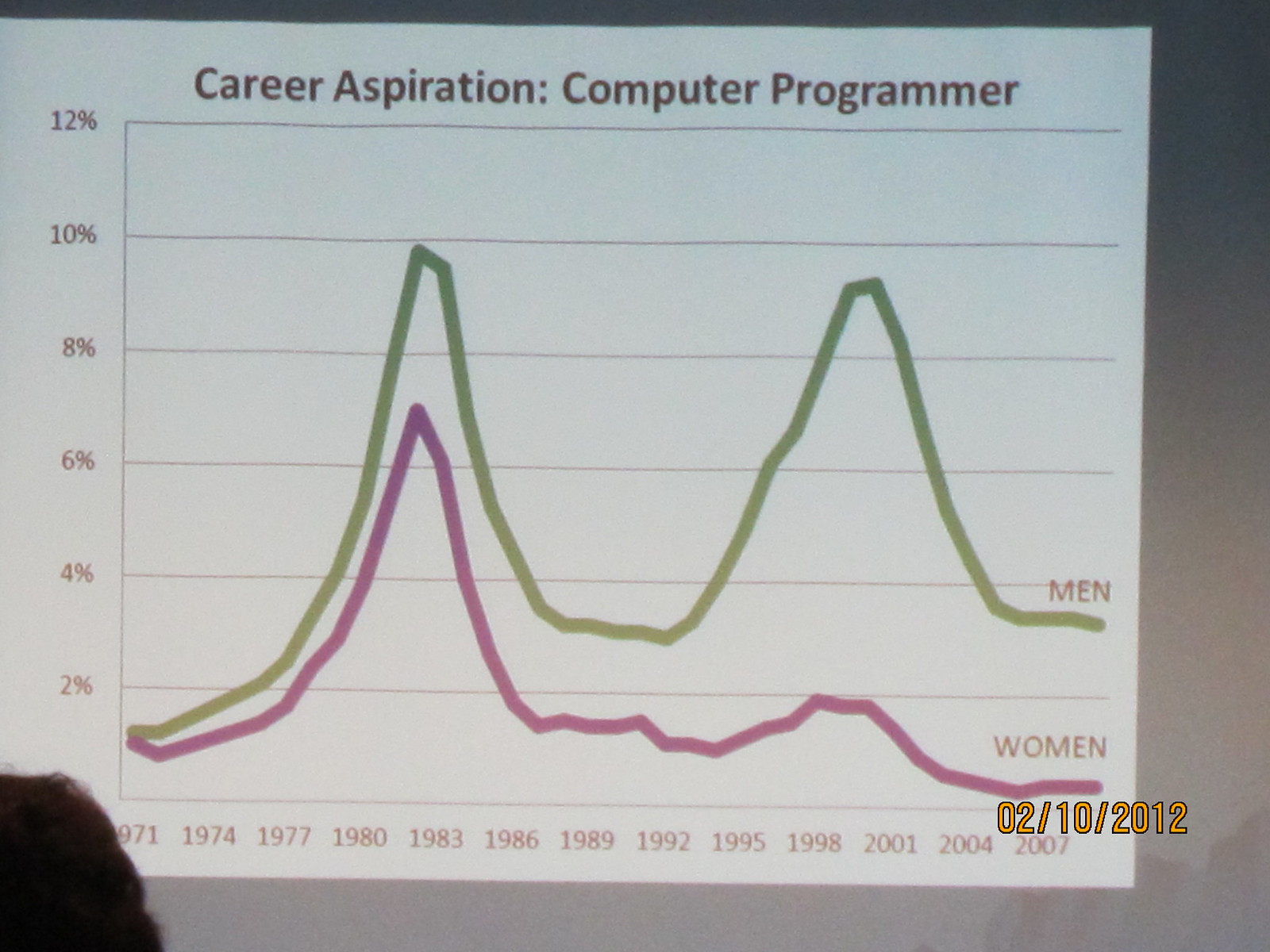The photograph, seemingly captured with a phone or digital camera on February 10, 2012, depicts a classroom or presentation setting. At the bottom left, there is a silhouette of a woman looking up at a central projection screen. The screen displays a slide titled "Career Aspiration: Computer Programmer," featuring a detailed line graph. The graph, spanning from 1971 to slightly past 2007, shows percentages in 2% increments ranging from 2% to 12%. The green line represents men's interest, which is consistently higher than women's, marked by a purple line. Notable trends include a significant spike around 1981-82, a decline, an increase around 1999, and another drop afterward. The color scheme of the image includes gray, white, black, green, purple, brown, and yellow, underlining the indoors, daytime academic atmosphere.